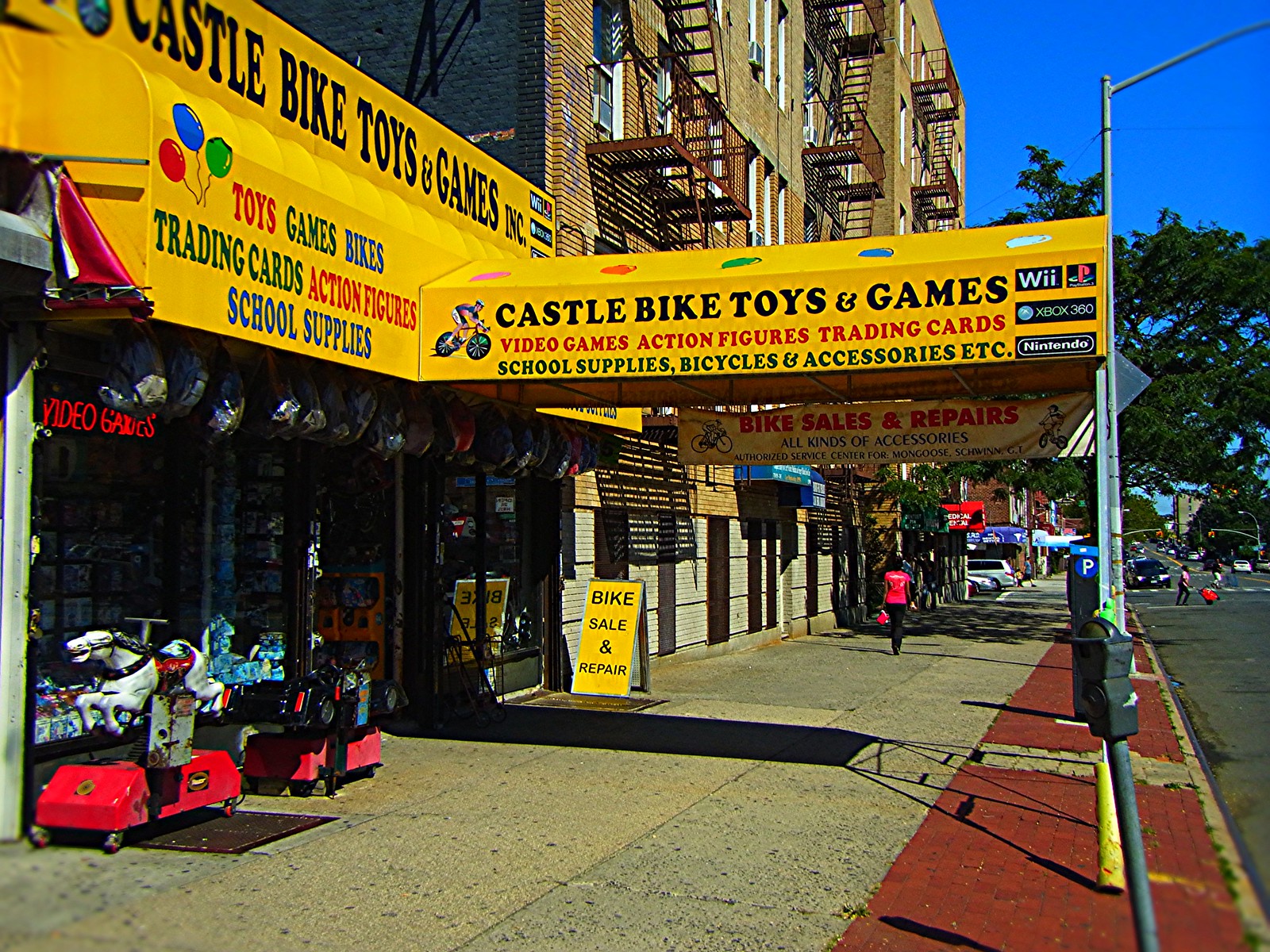This photograph captures a vibrant urban streetscape under a bright blue sky. Dominating the foreground is a lively store with a bright yellow sign and matching awning that reads "Castle Bike Toys and Games, Video Games, Action Figures, Trading Cards, School Supplies, Bicycles and Accessories" in a mix of black, red, green, and blue letters. The sign also features logos for Wii, PlayStation, Xbox 360, and Nintendo, alongside playful drawings including a man riding a bike, and colorful balloons that match the multicolored text. The storefront is bustling with activity; there are mechanical rides for children, including a rideable horse, as well as backpacks hanging outside. A neon sign in the window advertises Video Games in bright red letters. Additionally, a sign on the sidewalk promotes "Bike Sale and Repair." The sidewalk continues past the store, leading to old stone apartment buildings with visible fire escapes. On the right side of the frame, the bustling city street adds to the urban atmosphere, capturing the essence of daily life in this lively city area.